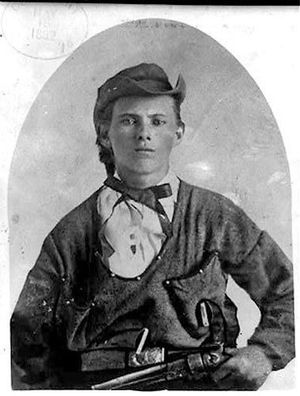This historical black-and-white photograph features a young man, likely from the 1800s, who presents a stoic and unmoving expression as he sits in a posed position. The image, which could be a tintype or daguerreotype, captures the essence of what might be a Wild West gunslinger or possibly a Civil War-era individual, though the attire does not specifically match any known soldier's uniform.

The man sports a frontward-facing old-fashioned hat with upturned corners and has a bit of long hair peeking out from underneath. He is dressed in a white button-down shirt with a darker vest layered on top, complimented by a black ribbon tied around his neck, resembling a bowtie. The shirt features a noticeable pocket sewn prominently on the front right.

Positioned across his lap, he holds a long-barreled revolver or rifle with his left hand, his right hand remaining out of sight. Around his waist rests a large, gleaming silver belt buckle that catches the eye amidst the otherwise monochromatic palette. This carefully staged photograph immortalizes a young man's semblance of the rugged and enigmatic figures of American history in a time long past.